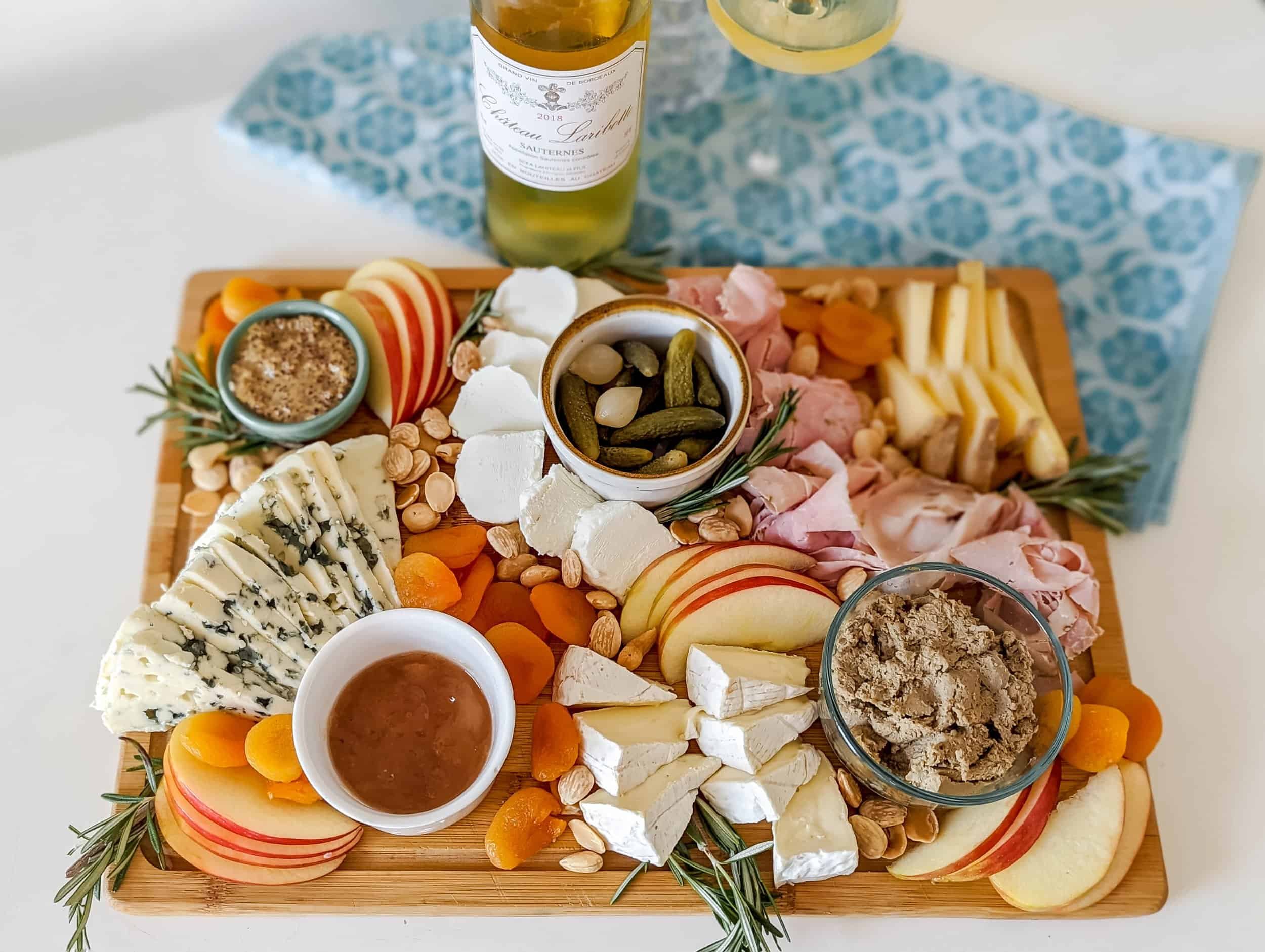The close-up photograph captures a meticulously arranged charcuterie board set on a large oak or bamboo cutting board, positioned horizontally and photographed from a three-quarters head-on angle. The array of delights on this horizontal board includes an assortment of pâtés, displayed in a small bowl, surrounded by bowls containing pickled garlic, gherkins, and various dips or preserves. In addition to the soft cheeses, such as brie and mozzarella, and slices of tangy blue cheese, the board boasts garnishes of rosemary twigs, thyme, and fine-sliced turkey lunch meat. Scattered throughout are dried apricots, sliced apples, and an assortment of nuts, including almonds and pistachios.

Behind this delectable selection, though slightly blurred, lies a teal and light teal-flowered cloth partially supporting a chilled bottle of white wine, adorned with an intricate, unreadable label written in cursive script. Nearby, the setup features a partially poured glass of the chilled wine, enhancing the overall elegant presentation of the charcuterie display.